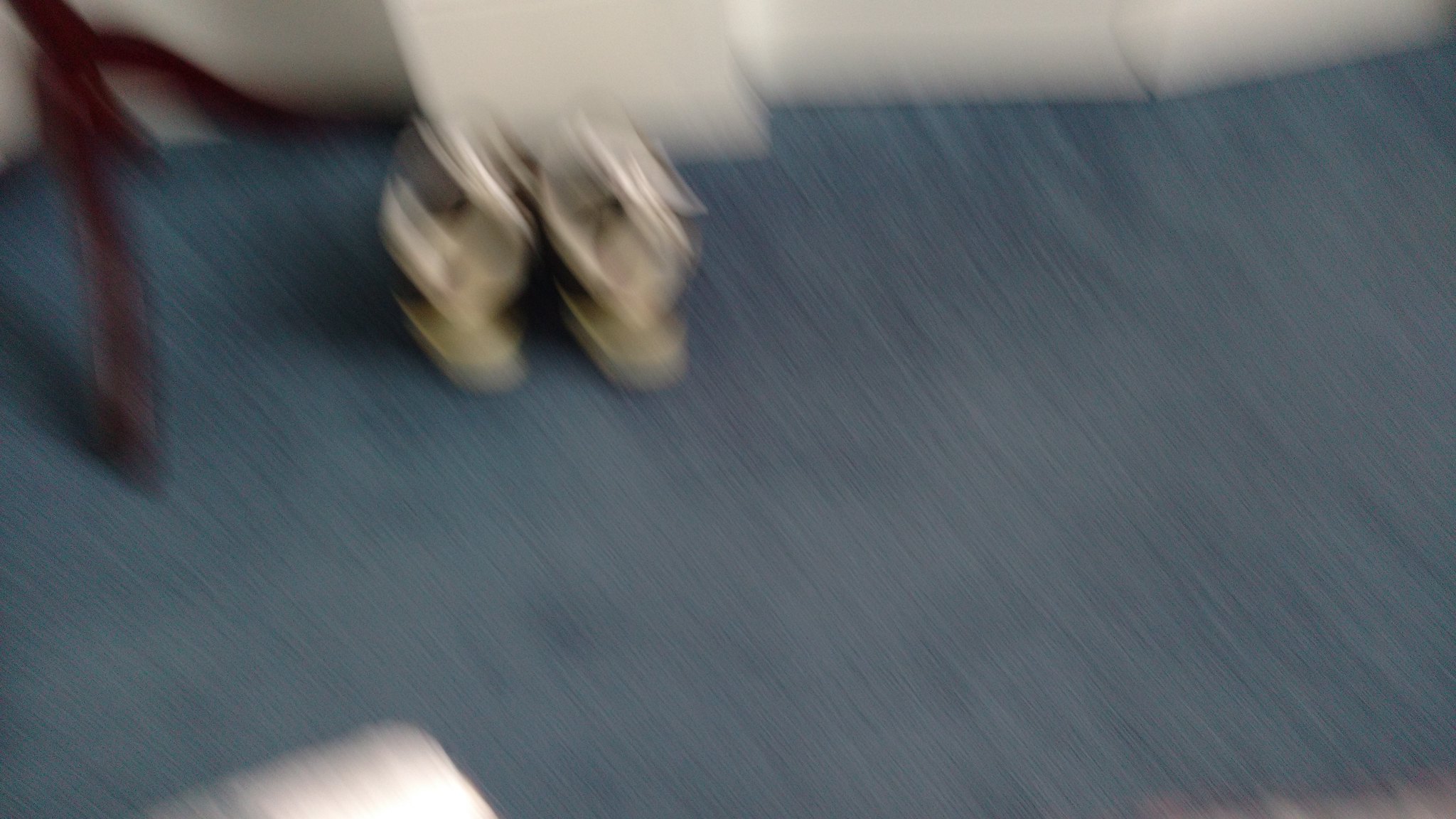This is a very blurry photograph taken with a shaky camera, capturing a scene pointing towards the floor. The image shows a plush blue carpet, likely the floor covering. Scattered across the carpet are a pair of shoes, which have a mostly white back, white on top, and black sides. In the upper right section of the image, there are what looks like three dark brown table legs. Additionally, there's a white object in the bottom left-hand corner, possibly the front of a couch, although it's difficult to distinguish due to the blurriness. The overall impression is of a hastily taken photo, not focused on any specific subject.